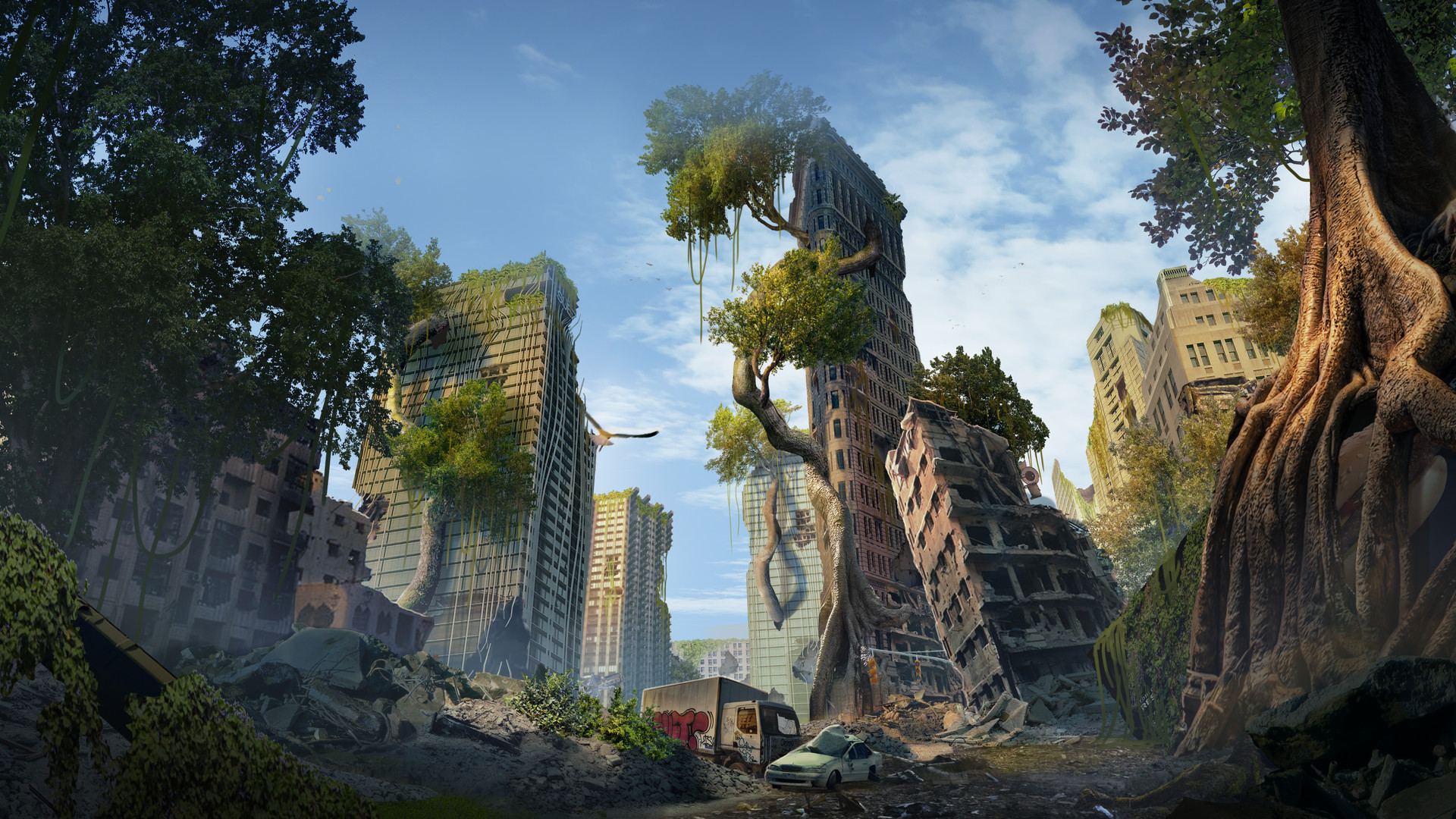This detailed drawing or digital art piece portrays a post-apocalyptic, dystopian cityscape where nature has reclaimed its territory over decaying urban structures. The scene is set under a blue sky with scattered clouds, juxtaposed against the crumbling remnants of skyscrapers, now overgrown with lush green plants. In the foreground, an abandoned street is strewn with rubble, featuring old trucks and cars with shattered windows, slowly succumbing to nature's takeover. The cityscape is dominated by two central, tall buildings that are visibly collapsed and broken, entwined with tree roots and vines. To the right, a large tree trunk rises majestically, leading up to dense green foliage, contrasting against the light gray, windowless buildings beneath. Additionally, a distinct triangular building with trees sprouting from its broken windows is leaning into another decrepit structure. On the far right, a massive tree wraps its roots over a rock, further emphasizing the fusion of nature and decay. In the distance, larger abandoned buildings loom, vacant and surrendered to the encroaching wilderness. This image vividly captures the eerie beauty of urban decay entwined with natural resurgence.